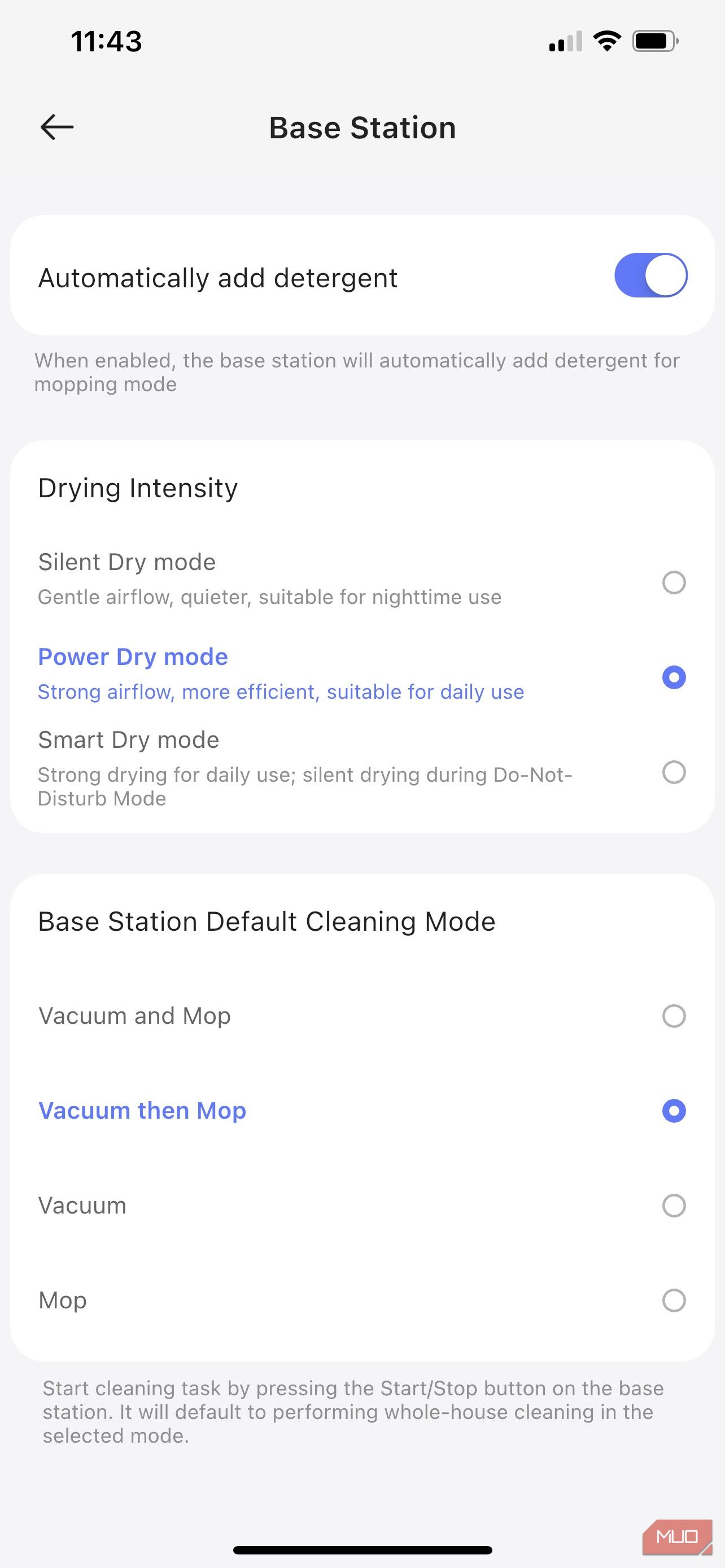This screenshot captures the settings page of a base station on a smartphone. The current time displayed at the top is 11:43. On the right side of the screen, there are icons indicating data bars, Wi-Fi signal strength, and battery life.

The first setting is a white box labeled "Automatically add detergent," with a toggle switch that has been turned on. Below, it describes, "When enabled, the base station will automatically add detergent for mopping mode."

The next section is titled "Drying Intensity," featuring three options:

1. **Silent Dry Mode**: Described as having gentle airflow for quieter operation, suitable for nighttime use.
2. **Power Dry Mode**: Highlighted in blue and currently selected, it features strong airflow for more efficient drying, ideal for daily use.
3. **Smart Dry Mode**: Alternates between strong drying for regular use and silent drying during Do Not Disturb mode.

Following this, there is another white box labeled "Base Station Default Cleaning Mode," providing four cleaning options:

1. **Vacuum and Mop**
2. **Vacuum then Mop** (currently selected and highlighted in blue)
3. **Vacuum**
4. **Mop**

Both "Power Dry Mode" and "Vacuum then Mop" are highlighted in blue, indicating that they are the active settings.